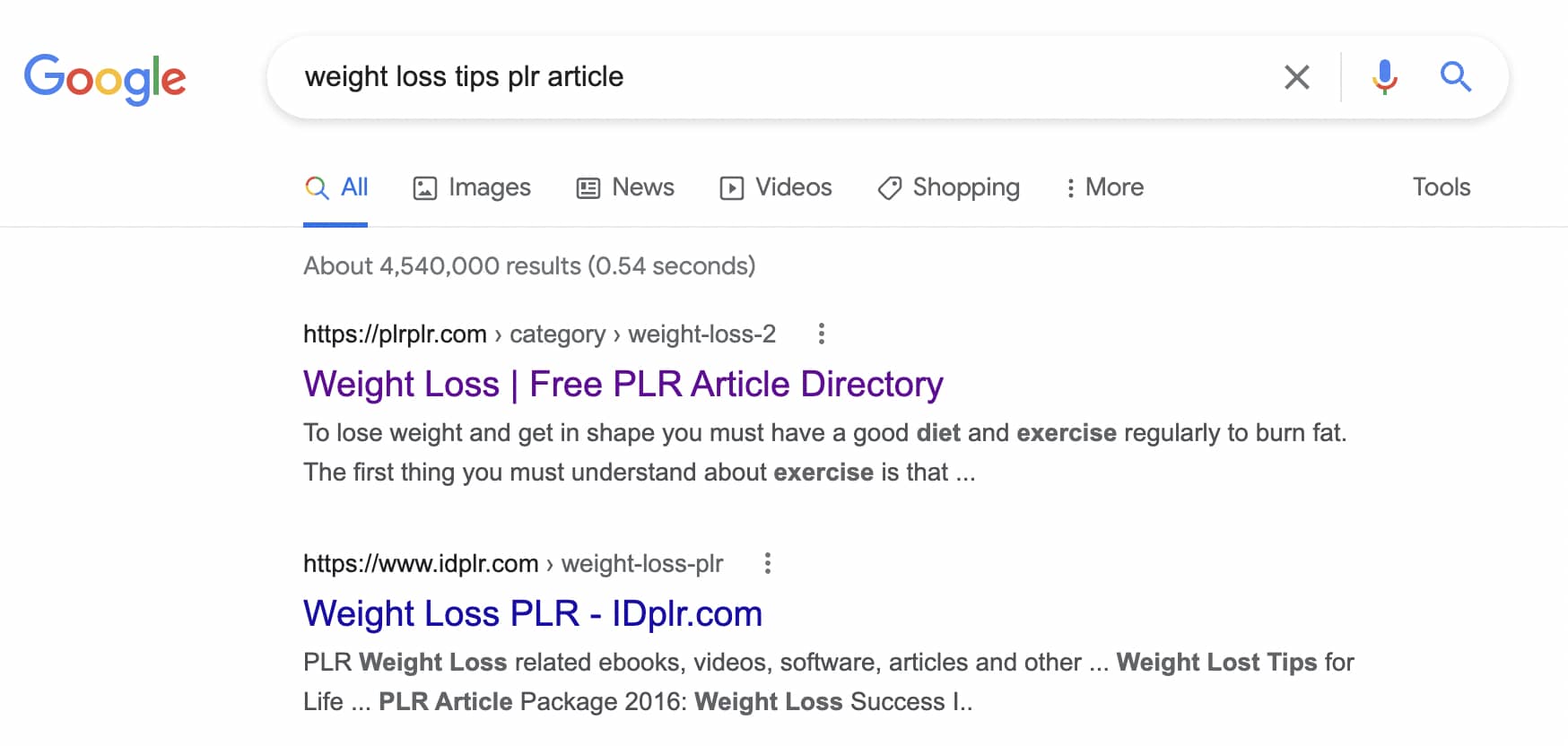This image is a cropped screenshot of a Google desktop web search page. Prominently displayed in the top-left corner is the Google logo. To its right is a search box containing the query "weight loss tips PLR article" typed in lowercase letters. Beneath the search box, the search results are partially visible. The first entry is a previously clicked link, shown in large purple text that reads "Weight Loss Free PLR Article Directory." Below this entry, another search result is visible, displayed in blue text with the website "weight loss PLR - LDPLR.com." 

Most of the additional search results are cropped out, limiting the view to the top portion of the page under the search bar, where categories such as "All," "Images," "News," "Videos," and "Shopping" are listed horizontally. The "All" category is selected. At the far right of these categories, in small gray letters, is the "Tools" option. To the right of the search bar, there is an 'X' to clear the search, a microphone icon for voice search, and a blue magnifying glass icon to execute the search. The overall webpage is characteristic of a standard Google search results layout.